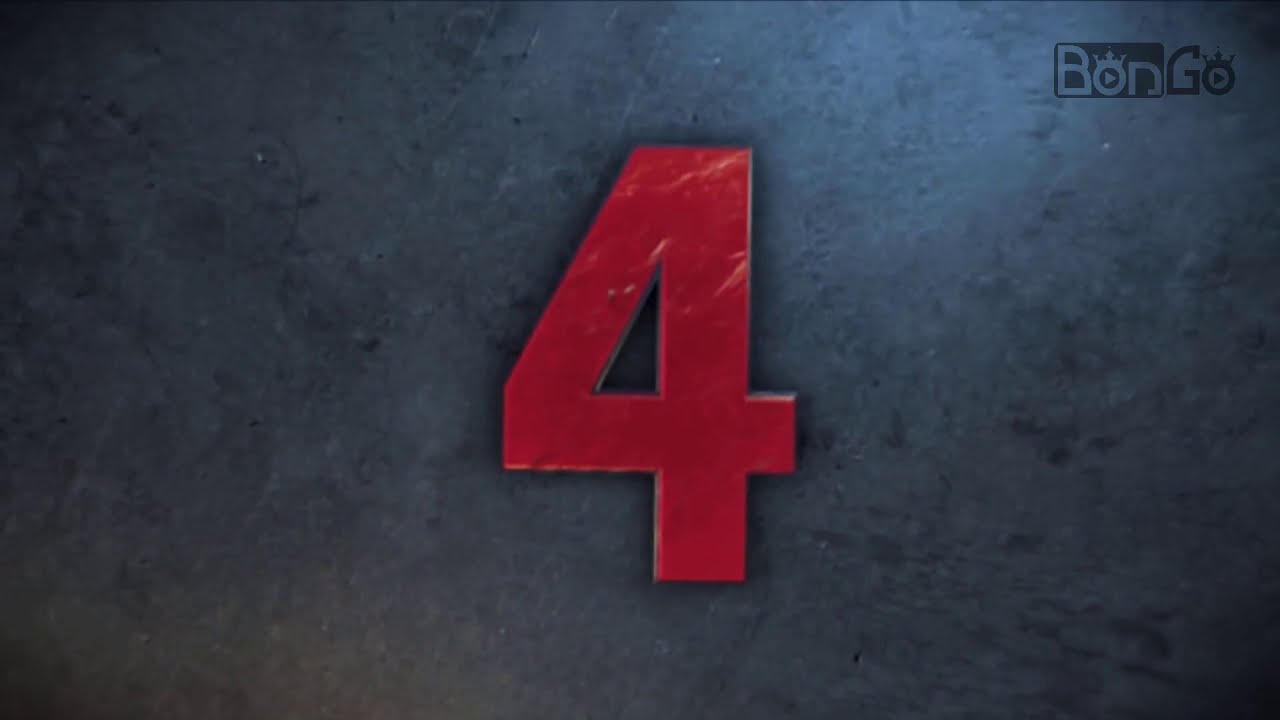The image features a highly stylized red number 4 prominently placed in the center against a dark, smoky gray and black marbled background. The number 4 has beveled edges with a drop shadow, and a marbly scratch texture with faint white lines running through it, giving it a weathered, three-dimensional appearance. The background transitions from light gray to darker shades with black specks scattered throughout, creating a worn, metallic surface effect. In the upper right-hand corner, there is a distinctive logo with the word "BONGO." The letters "BON" are displayed in a reverse font over a black rectangle, making the background image visible through the transparent text, while "GO" is presented in black letters. Both O's in "BON" and "GO" are uniquely styled with crowns and play button-like triangles above them.